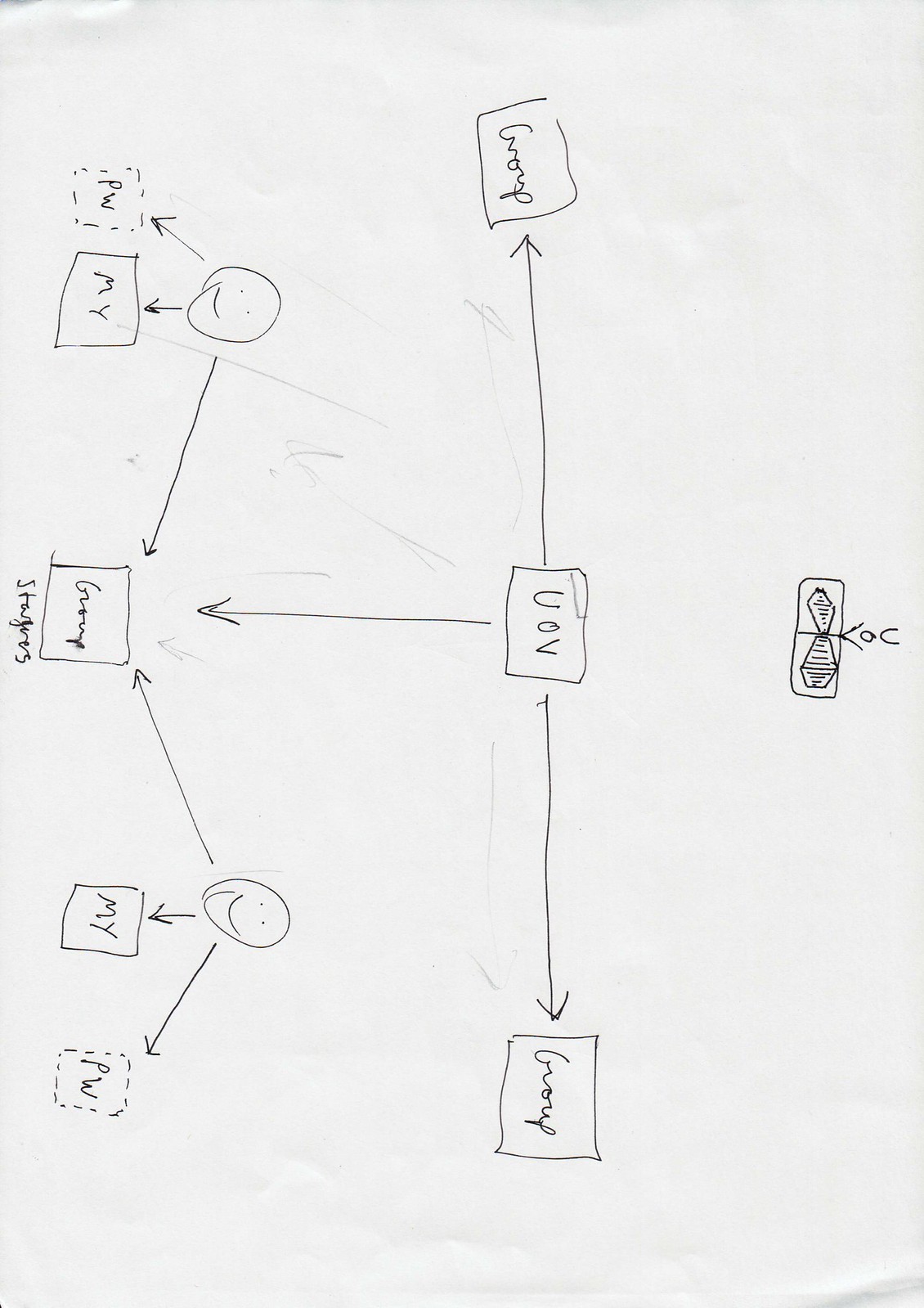This black-and-white photograph depicts a handwritten flowchart made with a black pen or pencil. The paper appears slightly crumpled, especially noticeable in the bottom left corner. The top left corner of the image has a gray edge, suggesting it might be slightly curved or the photograph may have been placed against a non-flat surface.

When rotating the image 90 degrees to the right, the flowchart begins with a square at the top, oriented like a diamond. This square contains a small stick figure, which has a circle for a head, two raised lines representing arms, and two lines for legs. This figure seems to be positioned as the starting point of the flowchart.

Beneath the stick figure, three rectangles are arranged in a row, each connected by arrows originating from the center rectangle. The left and right rectangles both contain the word "group," while the middle rectangle is labeled "UOV." 

A downward-pointing arrow links the middle rectangle to a series of additional rectangles. The central rectangle in this next row is also labeled "group," with the word "strangers" written below it. Positioned to the right of this arrangement, there is a round smiley face with an arrow pointing downwards to another rectangle labeled "my." Adjacent to this, a dotted-line rectangle labeled "PW" is positioned to the left.

Further to the right, another smiley face is connected by an inward-pointing arrow to the central "group" rectangle and also has a downward-pointing arrow leading to a rectangle labeled "my." This leads to another dotted-line rectangle on the right, labeled "PW."

The paper surface displays some indentations and smudges, though it is unclear whether these are actual marks on the paper or artifacts on the screen displaying the photograph.